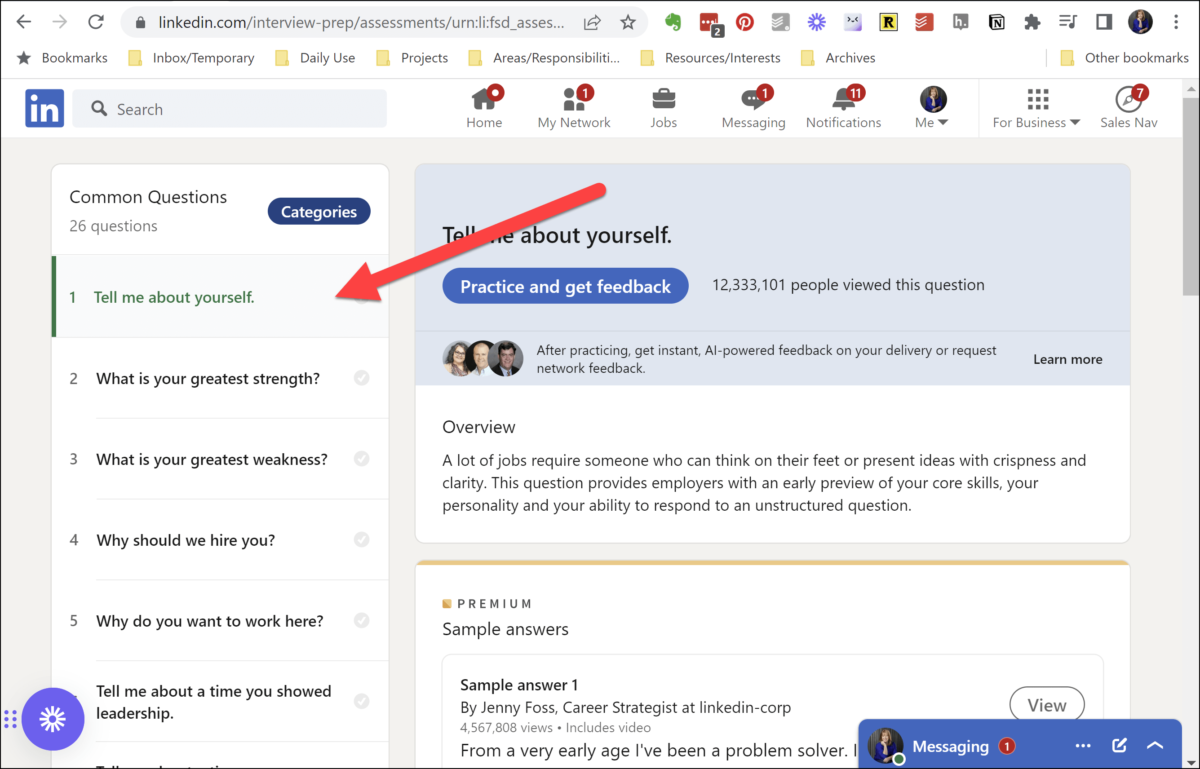The image is a screenshot of a LinkedIn interview preparation page. At the very top, there is a standard browser navigation bar displaying a variety of open tabs including icons for a fish, Pinterest logos, gearboxes, and several other icons, totaling around eight active tabs. This bar also includes commonly used controls such as a search button, a grayed-out forward button, a refresh button, and a back button.

Below this navigation bar, the user is signed into their LinkedIn account. The interface prominently features several bookmarks labeled "Inbox," "Temporary," "Daily Use," "Projects," "Error," "Responsibilities," "Resources," and "Archives." Additionally, there are other bookmarks listed towards the right end of this row.

The next row down highlights LinkedIn’s interface. On the left, the LinkedIn logo ("in") is visible in blue, accompanied by a search bar. To the right of the search bar, there is a series of icons labeled "Home" (currently marked with a red notification dot), "My Network" (depicted with two user silhouettes and a "1" indicating new activity), "Jobs" (illustrated with a briefcase icon), and "Messaging" (currently showing one new message). Furthermore, a bell icon signifies notifications.

Directly below the search bar, there is a section devoted to common interview questions. It includes a list numbering from one to six, illustrating frequently asked interview questions highlighted in green and red. The listed questions are:
1. "Tell me about yourself" (marked in red with a left arrow).
2. "What is your greatest strength?"
3. "What is your greatest weakness?"
4. "Why should we hire you?"
5. "Why do you want to be here?"
6. "Tell me about a time you showed leadership."

Adjacent to this list, on the right, is a blue box endorsing the "Tell me about yourself" question, encouraging users to practice and receive feedback. This section provides an overview of the question, demonstrates how many people have viewed it, and offers sample answers for practice.